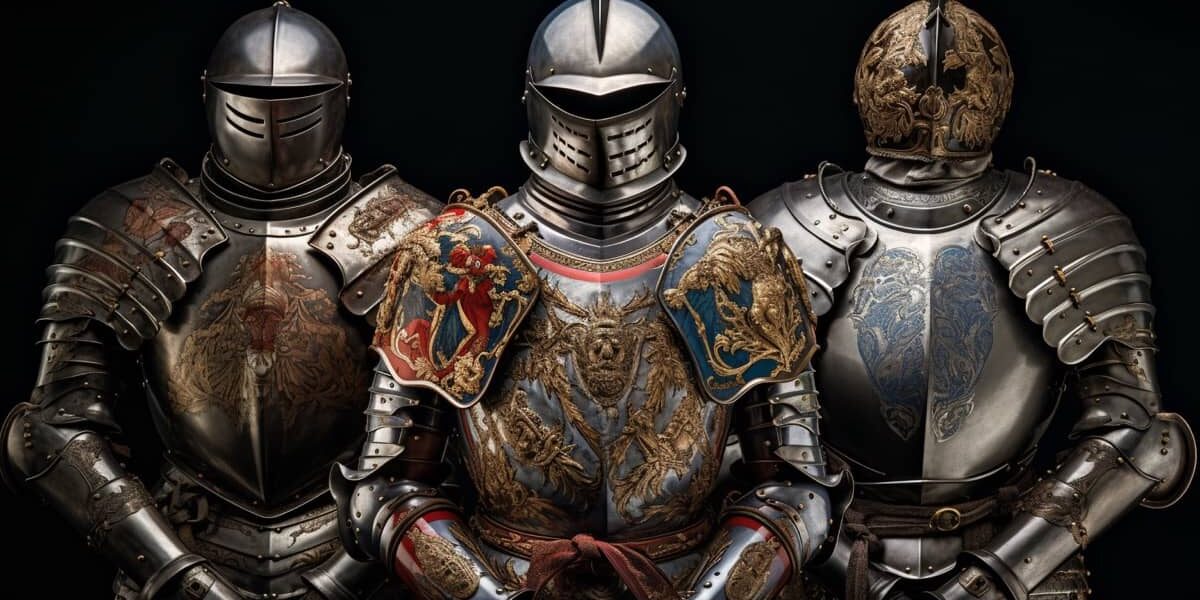The photograph captures a striking indoor scene set against an all-black background, showcasing three medieval suits of armor standing side by side. Each suit is made of metal, with intricate decorative designs that highlight their historic craftsmanship.

The suit on the left is a darkish silver, adorned with a small, indistinct brown painting on its chest, possibly of a dragon with its mouth open. The helmet is shiny but slightly tarnished, and the suit presents a strong, imposing figure.

In the center, the knight's armor features vibrant gold designs across its chest plate and elaborate blue, gold, and red motifs on the shoulder pads. It wears a distinctive red sash around its waist and has a crest that resembles a lion, adding to its regal appearance.

The suit on the right is predominantly silver with ornate gold details intricately decorating its helmet. The chest plate features blue filigree patterns, enhancing its elegance. This suit also has a grayish belt around the waist, completing its refined look.

These meticulously crafted suits of armor, possibly from a medieval history museum, transport viewers back to the Middle Ages, evoking images of knights in shining armor ready for battle.